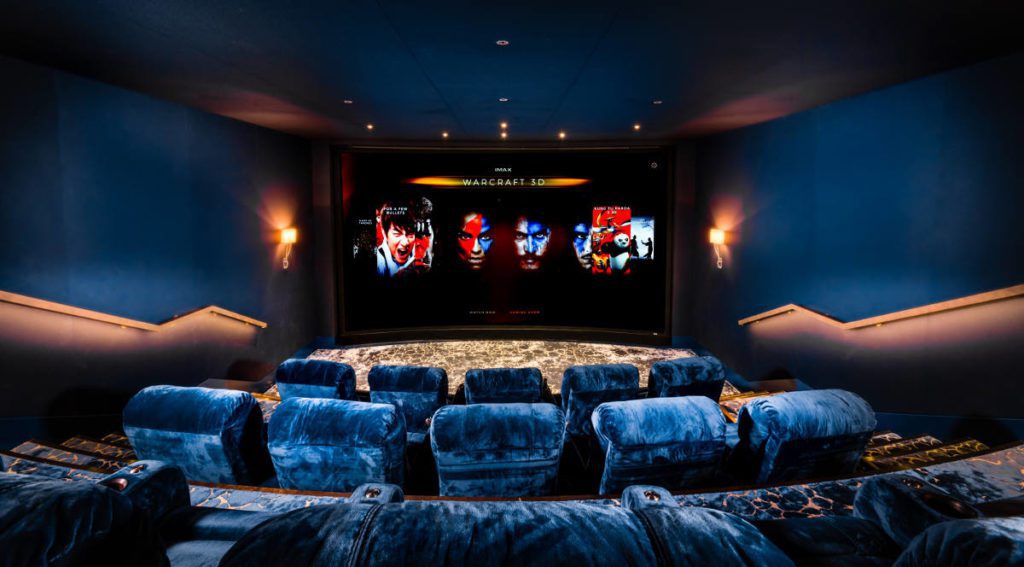This image showcases an elegant home theater. The room is bathed in calming blue hues, from the slightly angled blue walls to the blue ceiling featuring recessed white lighting. The ceiling's illumination gives the room a welcoming glow. The seating arrangement consists of three rows of plush, soft, blue velour or velvet upholstered seats, all equipped with cup holders in the armrests. The front of the room features a large, slightly curved screen displaying the introductory scene of "Warcraft 3D," with four characters visible – Kung Fu Panda on the right and another figure resembling Jackie Chan on the left. The carpeted steps sport a blue design with gold accents. The floor towards the screen appears two-toned, predominantly black and beige or gray, creating a multi-colored visual effect. The entire setting exudes luxury and comfort, perfect for an immersive movie-watching experience.